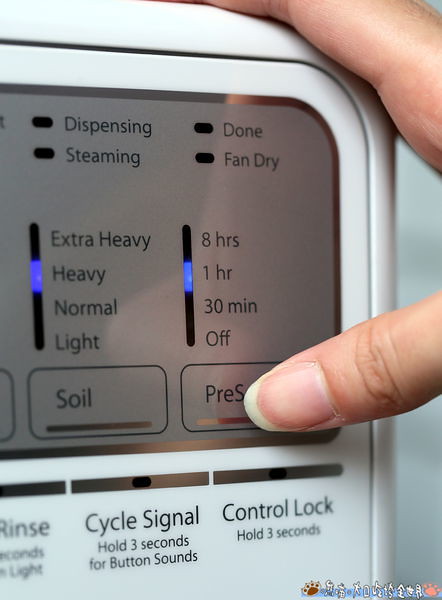This is a detailed photograph of someone operating a washing machine's white control panel. The control panel features options categorized by blue vertical lines on both the left and right sides to indicate different settings. On the right side, the options include "8 hours," "1 hour," "30 minutes," and "Off," while on the left, the settings are "Extra Heavy," "Heavy," "Normal," and "Light." Below these options, the panel includes several buttons to control various functions: the first button's label is not visible, but the subsequent buttons are labeled "Soil," "Pre-Soak," "Rinse," "Cycle Signal," and "Control Lock." The "Control Lock" must be held for three seconds to activate. All the text on the machine is in black, and the hand shown in the upper right corner is pressing buttons, interacting with the machine's touchscreen interface.